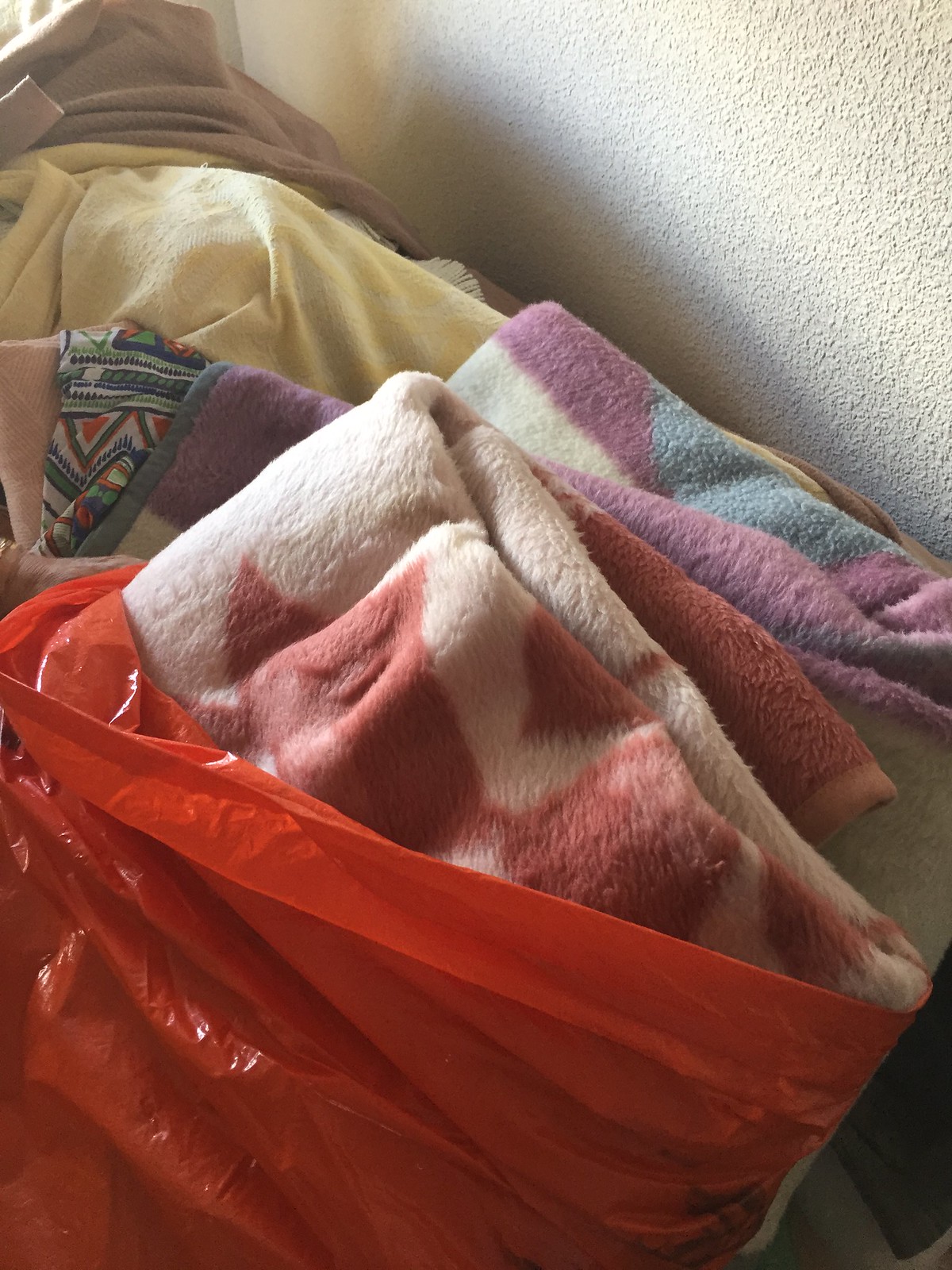This color photograph captures a scene featuring a prominent red plastic shopping bag with a tomato-red hue, displaying a slight tinge of orange. The bag appears crinkly and is situated coming up from the bottom left corner of the image. Inside the bag, two folded, fluffy blankets with a soft texture are visible. The top blanket is light pink with darker pink markings, while the one beneath it is white with hints of blue and dusty purple shades, both folded into neat rectangles.

To the side of the bag, there is a disordered pile, possibly of laundry, including various items such as tan fabric with some yellowing and a darker brown item behind it. This heap of fabric is positioned in the top left-hand corner of the image.

In the background, a white wall with a heavily textured, popcorn ceiling-like finish provides a backdrop. Natural sunlight illuminates the scene, casting shadows and highlights across the blankets and the wall. This lighting accentuates the textures and folds in both the plastic bag and the soft, fuzzy fabrics within it.